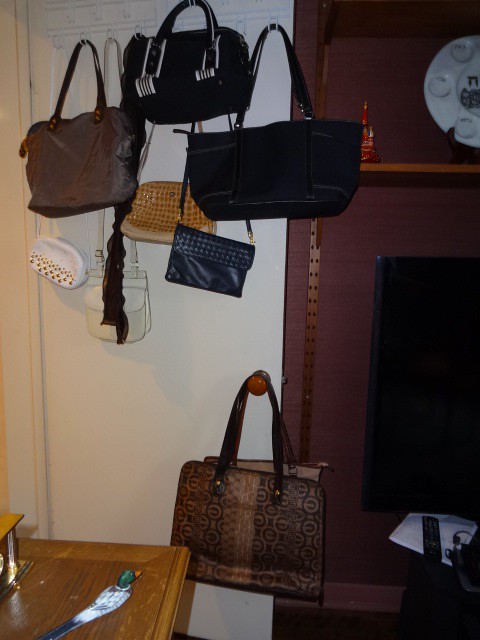This photograph captures a cozy interior room, dominated by a white door adorned with an assortment of purses and bags. The door, featuring a brown wooden doorknob, has a total of eight handbags hanging from hooks at its top and a prominent mosaic-patterned bag attached to the doorknob. The purses vary in style and color: there’s a dark brown purse with a lighter brown stripe, a black rectangular bag with two side pockets, a black purse with white piping, a brown-gray handbag, a small white over-the-shoulder bag with gold metal detailing, an off-white oval-shaped bag with a large front pocket, a tan animal-skin patterned bag, and a dark blue handbag with lighter blue metal accents. 

In the foreground on the left, a light brown wooden table hosts a charming statue of a mallard duck. The background on the right reveals a slice of a dark burgundy wall, partially obscured by the edge of a television screen. Below the television, some papers and a remote control are scattered. Two shelves held up by a metal brown bracket are also visible on the wall. The detailed background and assortment of purses give the room a lived-in, eclectic feel.